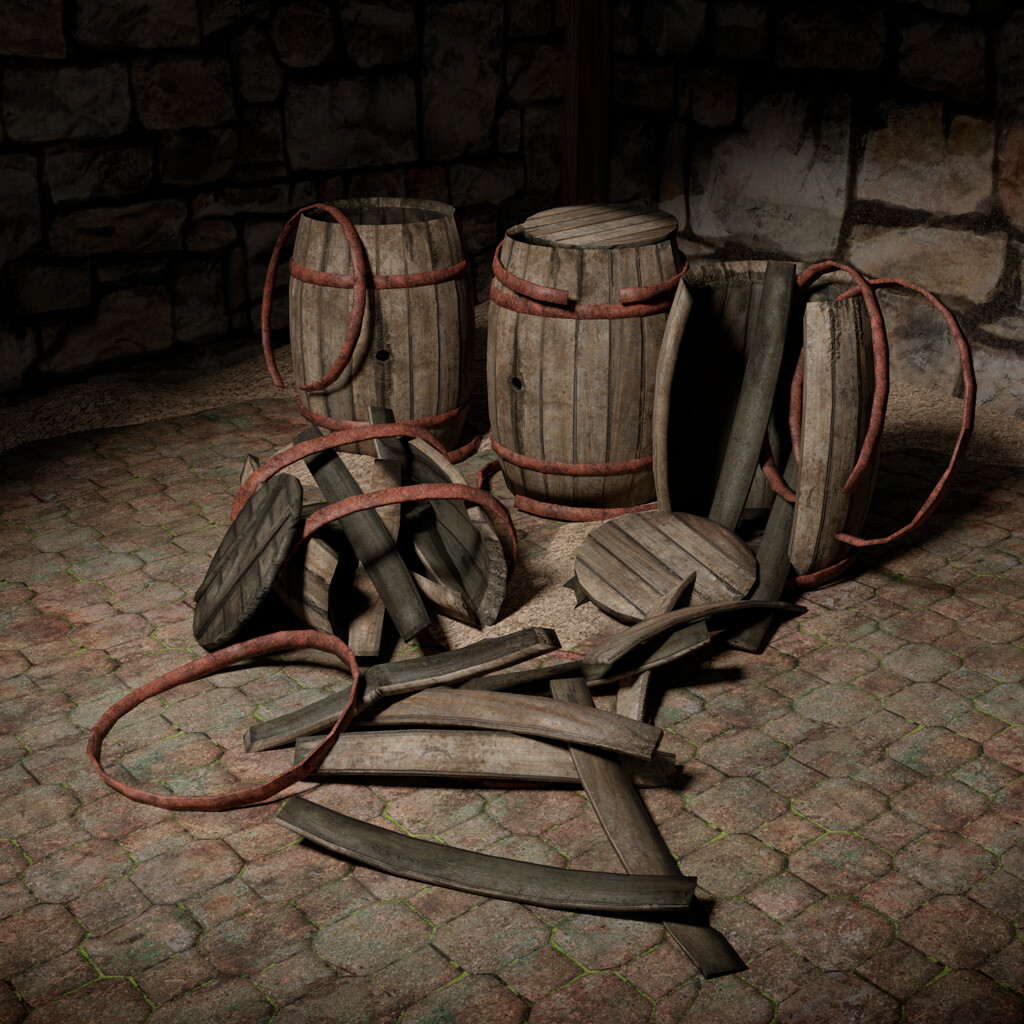In a dimly lit, atmospheric cellar with shadowy corners, this color photograph captures the scene of several old wooden barrels in various states of condition on a cobblestone floor. The cellar's stone walls and dark environment envelop the scene in shades of orange, brown, black, and gray. Three barrels stand upright; the one on the left is missing its top with a rusted ring loosely hanging off its lip, while the one in the center is intact and complete with a wooden top. The third upright barrel is partially constructed, with side slats still needing to be assembled, and nearby are scattered barrel parts, including brass hoops and wooden slats. In front of these, the shattered remains of a fourth barrel lie in pieces on the cobblestones, adding to the rustic, historic feel of the scene. The distinct red rings on some of the barrels provide a pop of color amid the earthy tones. The detailed setting evokes a bygone era, perhaps suggesting the barrels were once used for aging wine or spirits.